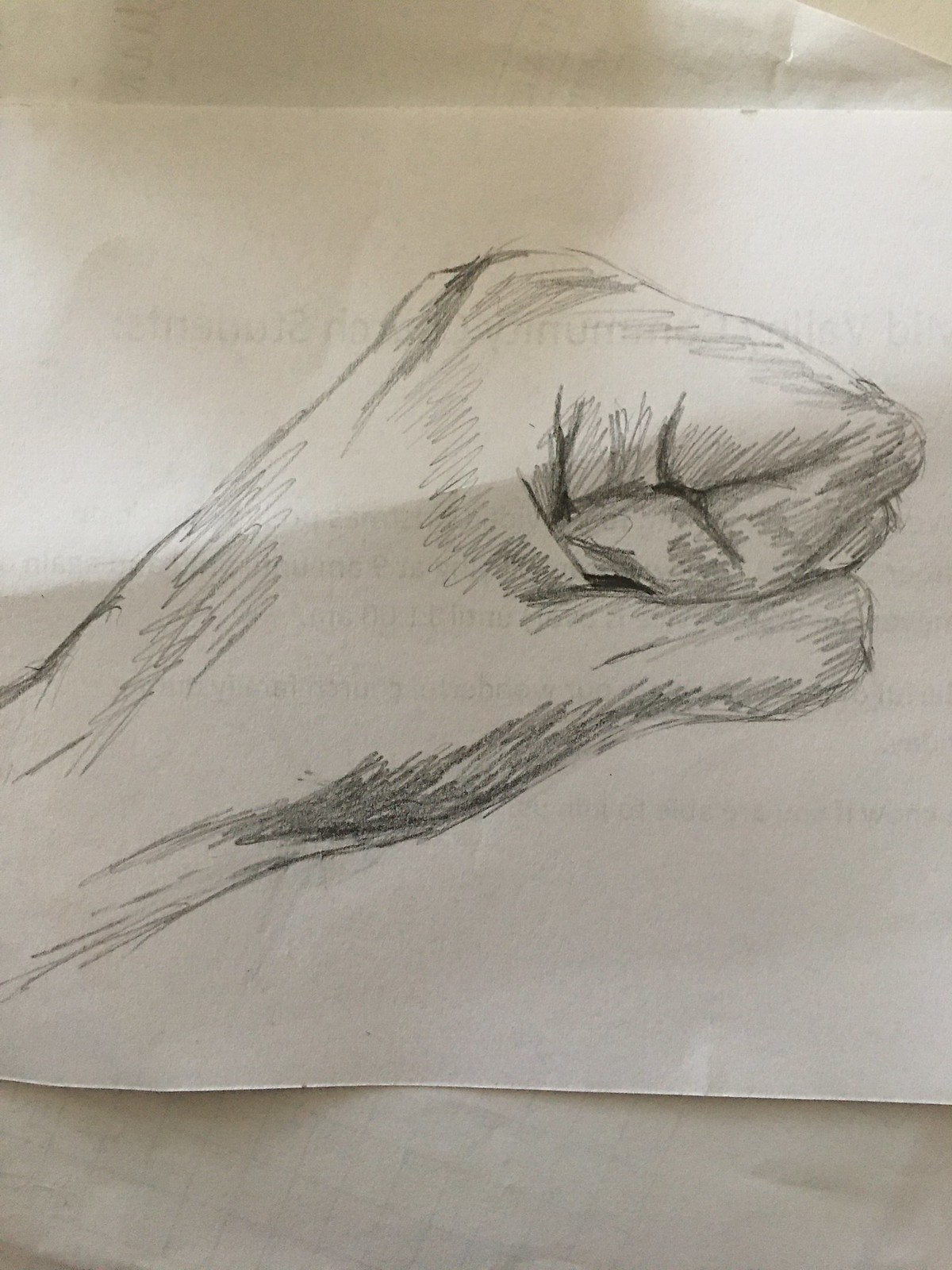A detailed pencil drawing on a plain, unlined piece of copy paper. The drawing itself depicts a left-handed fist, angled from the lower left towards the upper right corner of the paper. The thumb is tucked beneath the closed fingers, representing a tightly clenched fist. The artwork features bold, prominent outlines that emphasize the outer edges of the hand, as well as the areas of tension where the fingers bend and crease. These additional lines accentuate the strain and realism of the clenched fist. The background is simple, consisting of another sheet of unlined copy paper beneath the drawing, creating a minimalistic backdrop that highlights the detailed pencil work.